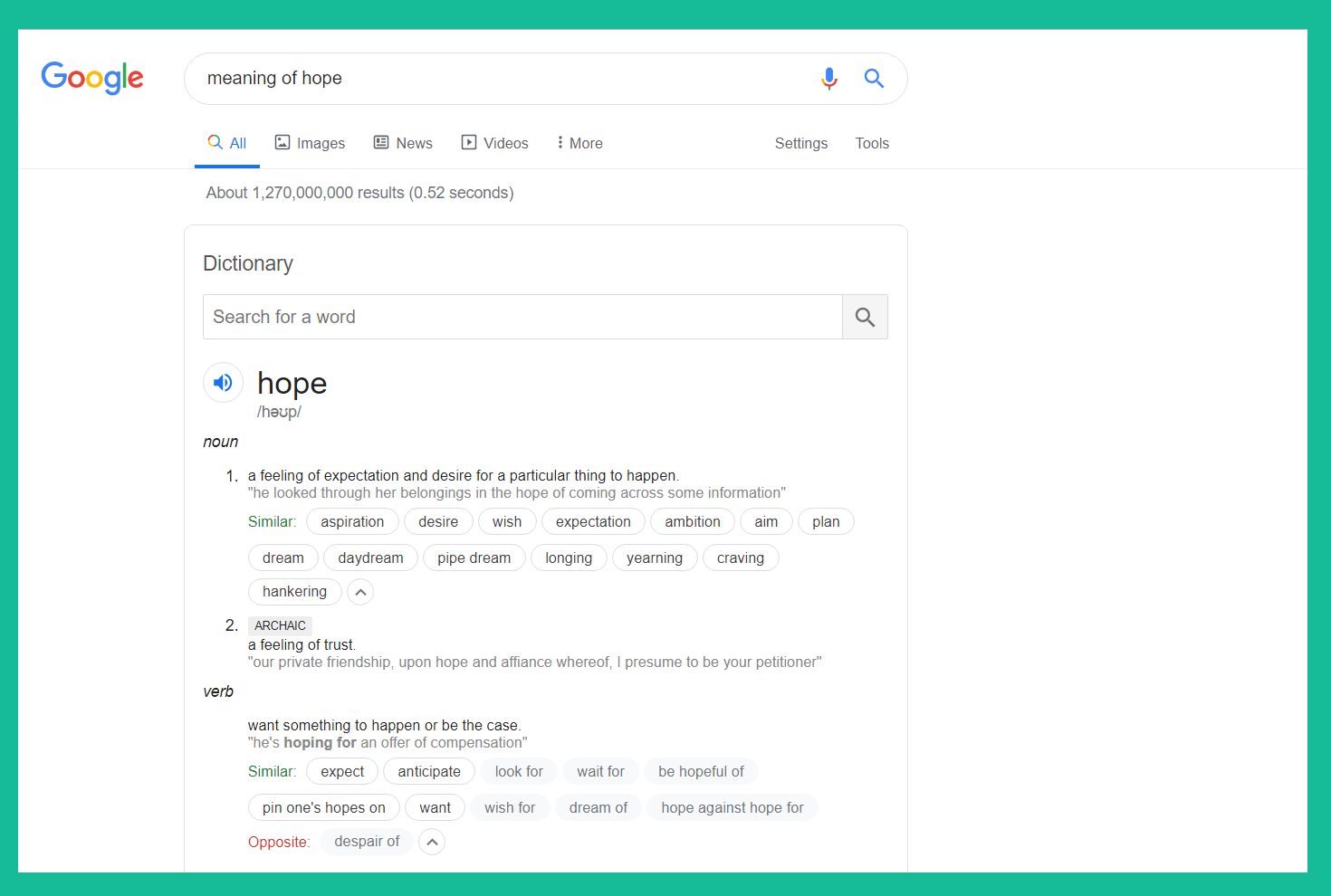The image is a screenshot with a green border and a white background. In the upper left corner, the Google icon is prominently displayed. To the right of the icon, there is a search bar containing the text "meaning of hope," along with icons for the Google microphone and a magnifying glass. Below this, there are navigational options including "All," "Images," "News," "Videos," "More," "Settings," and "Tools," all outlined in light gray.

Further down, the word "Dictionary" is highlighted. Underneath, another search bar with a magnifying glass is visible. Below this bar, the word "hope" is displayed in bold, accompanied by a small speaker icon presumably for audio pronunciation of the word. The entry classifies "hope" as a noun and provides the following definition: "A feeling of expectation and desire for a particular thing to happen. Example: He looked through her belongings in the hope of coming across some information."

Additionally, the definition includes similar words: aspiration, desire, wish, expectation, ambition, aim, plan, dream, daydream, and pipe dream.